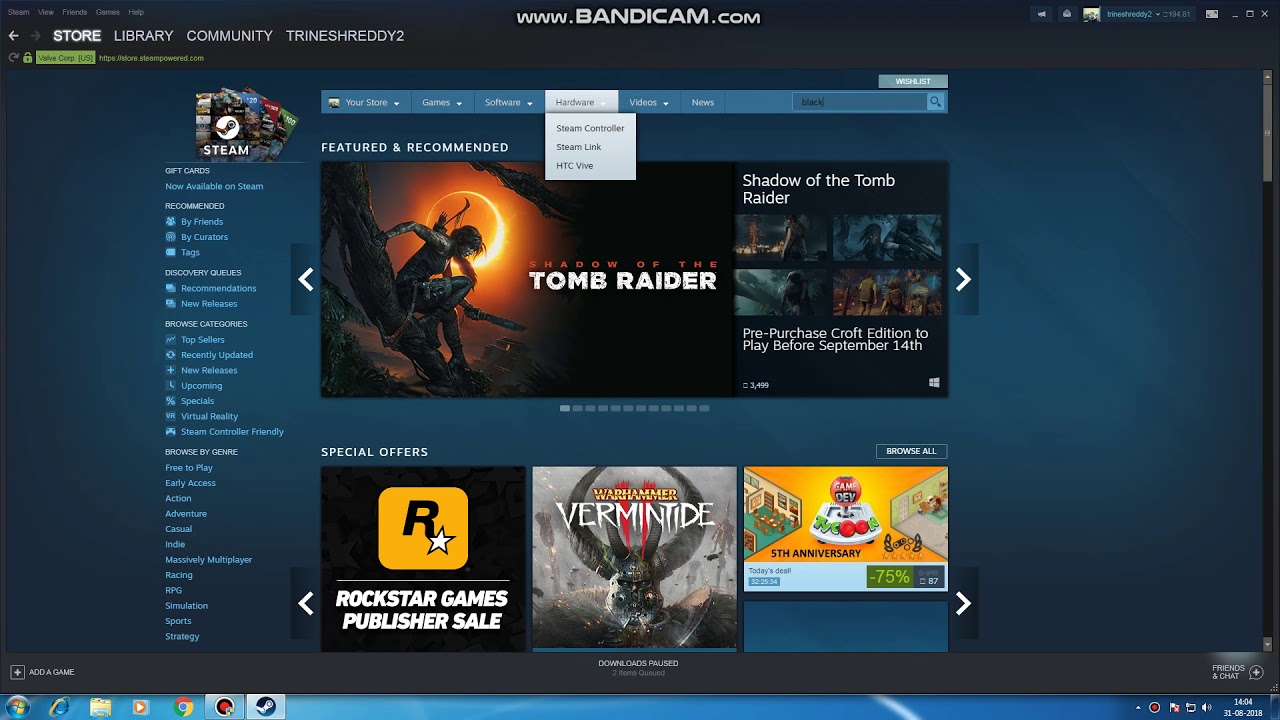The image depicts a computer screen with a predominantly blue background flanked by black borders on the top and bottom. The very bottom features a blue border. In the upper left corner, the screen displays white text reading "Store," "Library," "Community," and "Train Shreddy." Centered at the top is the URL "www.bandicam.com."

In the center of the screen, there is a prominent display of video games. The highlighted game is "Shadow of the Tomb Raider," featuring the iconic Tomb Raider character. The cover art shows the character sitting on what appears to be a tree root, with a celestial body, possibly the sun or moon, illuminating the background. The cover predominantly uses shades of black and has a mysterious ambiance.

Adjacent to the Tomb Raider game cover is a navigational menu, predominantly blue with main sections outlined in white. Below the highlighted game, other games are displayed. One of the recognizable publishers is Rockstar Games. To the right of this, the game "Vermintide" is visible, while the title of another game next to it is unclear.

At the bottom of the screen on the blue banner are several logos, including the Microsoft logo, a browser logo, and the Google Chrome logo. On the right side, the time is displayed, although it is not legible in the image.